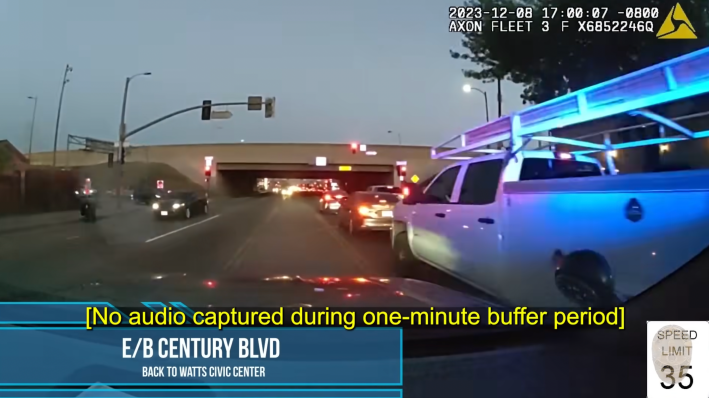The image, likely a screenshot from a television or a police car camera, captures an evening traffic scene on eastbound Century Boulevard heading back to Watts Civic Center. The forefront includes a white utility pickup truck with a rack on top in the right lane, amidst heavy traffic. Additional vehicles, including some with their headlights on, are seen traveling in both directions. A prominent red streetlight hangs above the scene, while a brown overpass stretches horizontally across the center. On the lower part of the screen, a chyron reads "E/B Century Boulevard, back to Watts Civic Center," accompanied by the message "(No audio captured during one minute buffer period)" in yellow text. The bottom right corner features a speed limit sign of 35 mph. The top right corner displays the timestamp "2023-12-08 17:00:07/08, Axon Fleet 3 FX6852246Q" in white text.